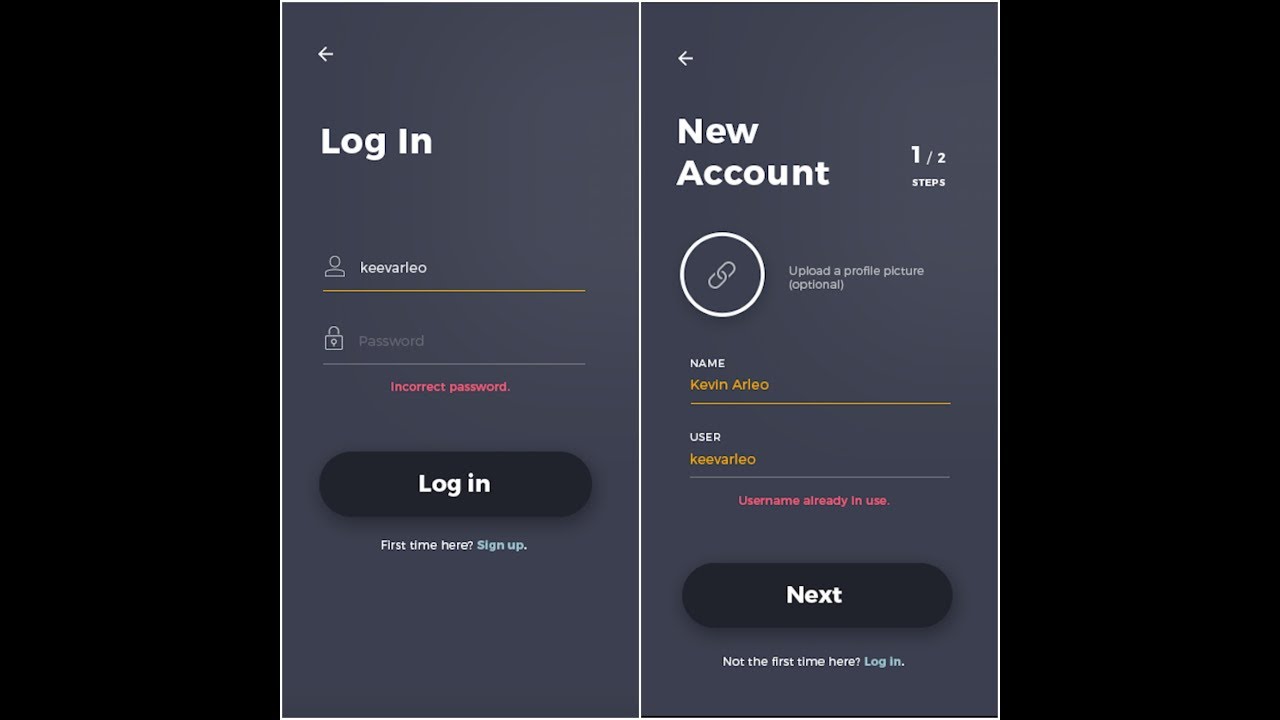The image consists of four rectangular boxes arranged horizontally. The sequence starts with a black box on the far left, followed by a gray box, another gray box, and ends with a black box on the far right.

In the first gray box:
- An arrow pointing left is depicted at the top, accompanied by the text "Log In".
- The text "Kiva Kiber Leo" appears prominently within the box.
- Below that, the field "Password" is shown, followed by a warning message "Incorrect password".
- Additional options provided include "Log In" and "First time here? Sign Up".

In the second gray box:
- The header reads "New Account".
- It mentions "One and a half steps" as the progress indicator.
- A circular icon resembling a paper clip is included, labeled "Upload a profile picture (optional)".
- The name "Kevin Arleo" is displayed.
- The username field shows "Kev Arleo" with a notification "Username already in use".
- Navigation options are "Next" and "Not the first time here? Log In".

Two black boxes flank either side of the gray boxes, adding a contrasting visual.